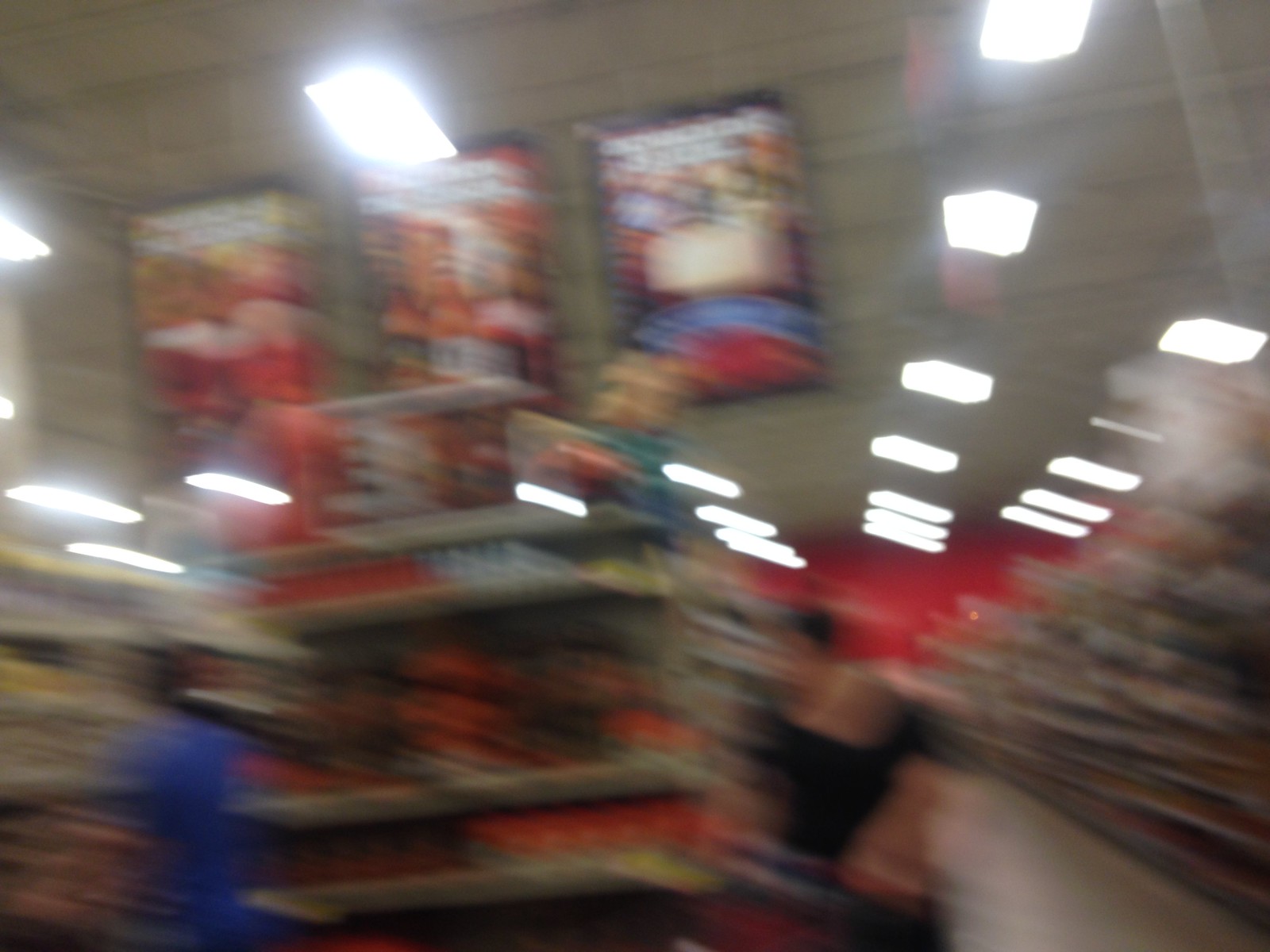This indoor photograph captures a scene within a commercial building, likely a Target store, given the distinctive red wall visible in the background. The image, although extremely blurry, shows the end caps of several aisles under the glow of fluorescent lighting. On the left, a person is seen wearing a cobalt blue shirt. To the right, another individual, likely a woman with short dark hair, is discernible, dressed in an outfit that appears black and tan, accented with white collars and cuffs. The off-white colored floor of the building is also visible, subtly reflecting the overhead lights.